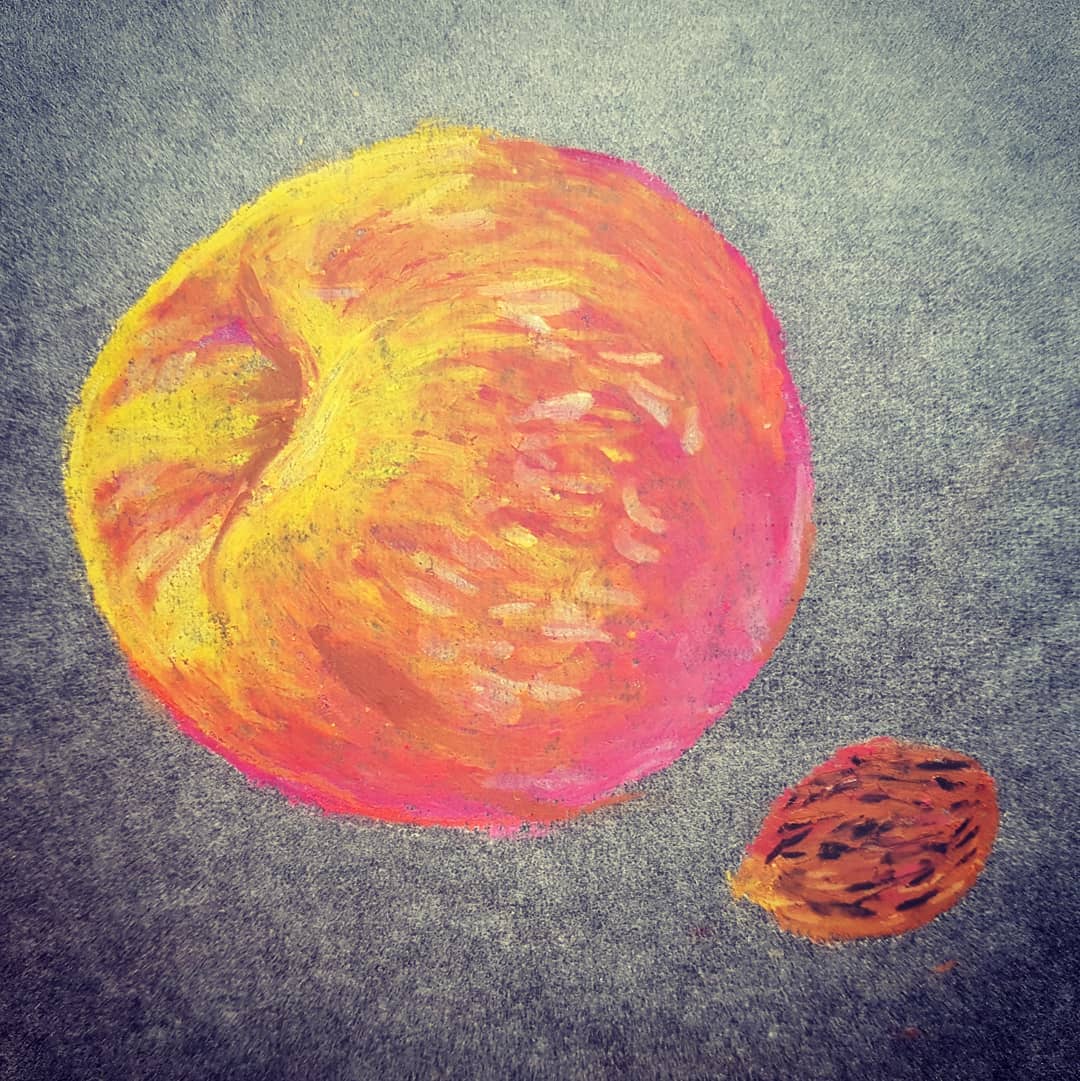This vibrant, color image is a semi-abstract painting set against a textured grey background that gradually shifts from lighter tones at the top to darker shades in the bottom corners. The background features a grainy texture, adding a subtle depth to the composition. Dominating the left side of the painting is an abstract depiction of a fruit, likely an apple or a peach. The fruit is vividly rendered with hues of yellow, red, and a delicate pinkish tint towards the right side. There is no discernible stem or seeds, allowing the viewer's focus to remain on the interplay of colors and shapes. Near the bottom right corner, a smaller, round object emerges, composed of seemingly scribbled lines in shades of brown, pink, yellow, and black. This object, somewhat resembling a nut, adds an intriguing and ambiguous element to the painting, inviting viewers to ponder its identity and significance. The overall effect is a captivating blend of color, texture, and abstract form.